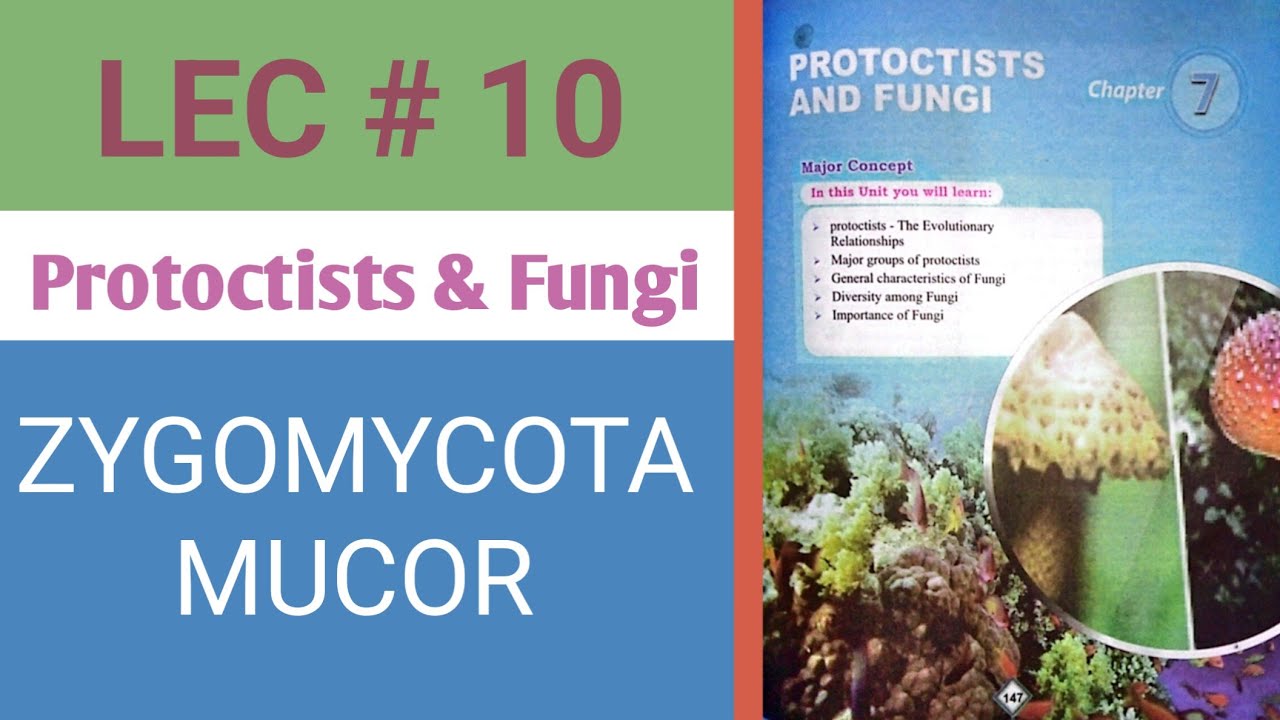This horizontal rectangular image appears to be an advertisement slide or card for a lecture or textbook chapter on protoctists and fungi, identified as lecture number 10. The top left corner features a green band with purple writing stating "Number 10", followed by a white band that reads "Protoctists and Fungi". Beneath this white band, a larger blue rectangle contains white lettering that says "Ivote Mycota Macrur". The right side of the image is divided vertically, reiterating the title "Protoctists and Fungi", with some small, illegible text next to it. Below this text, there is a white area with black print, also too small to read, and an illustration showing some fungi. The image seems to relate to a chapter in a science textbook, likely aimed at advanced high school or early college students, covering evolutionary relationships, major groups, general characteristics, diversity, and the importance of fungi within the biological domain.